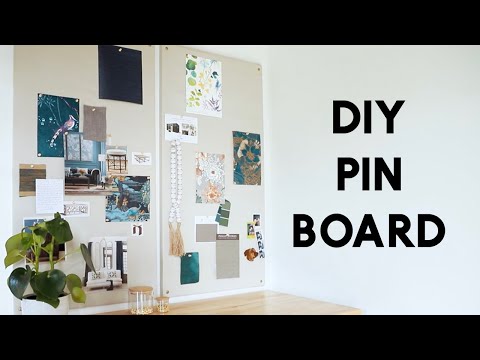The image depicts a corner of a room with wooden floors, showcasing an online ad for a DIY pinboard. The white wall features the black, capitalized lettering "DIY Pinboard" prominently across the top. Below this text, there are two large pinboards that span much of the wall, each adorned with various items. The right pinboard includes a floral design paper at the top, several paint samples, and a black sheet of paper pinned to it. It also features a picture of a living room with a blue wall and white lamp, a necklace with tan tassels, and a map in blue, tan, and gray hues. The left pinboard holds a dark background image of a bird, a notepad, a painting of a tropical scene with plants, and more eclectic content. 

In front of these boards is a light tan table, on which sits a potted plant with green leaves in a white planter and two small containers, one larger than the other, with wooden tops. Hanging from one of the boards are beads with a brush-like ornament at the bottom. The scene is framed by thick black lines at the top and bottom, completing the aesthetic of a carefully curated, creative workspace.